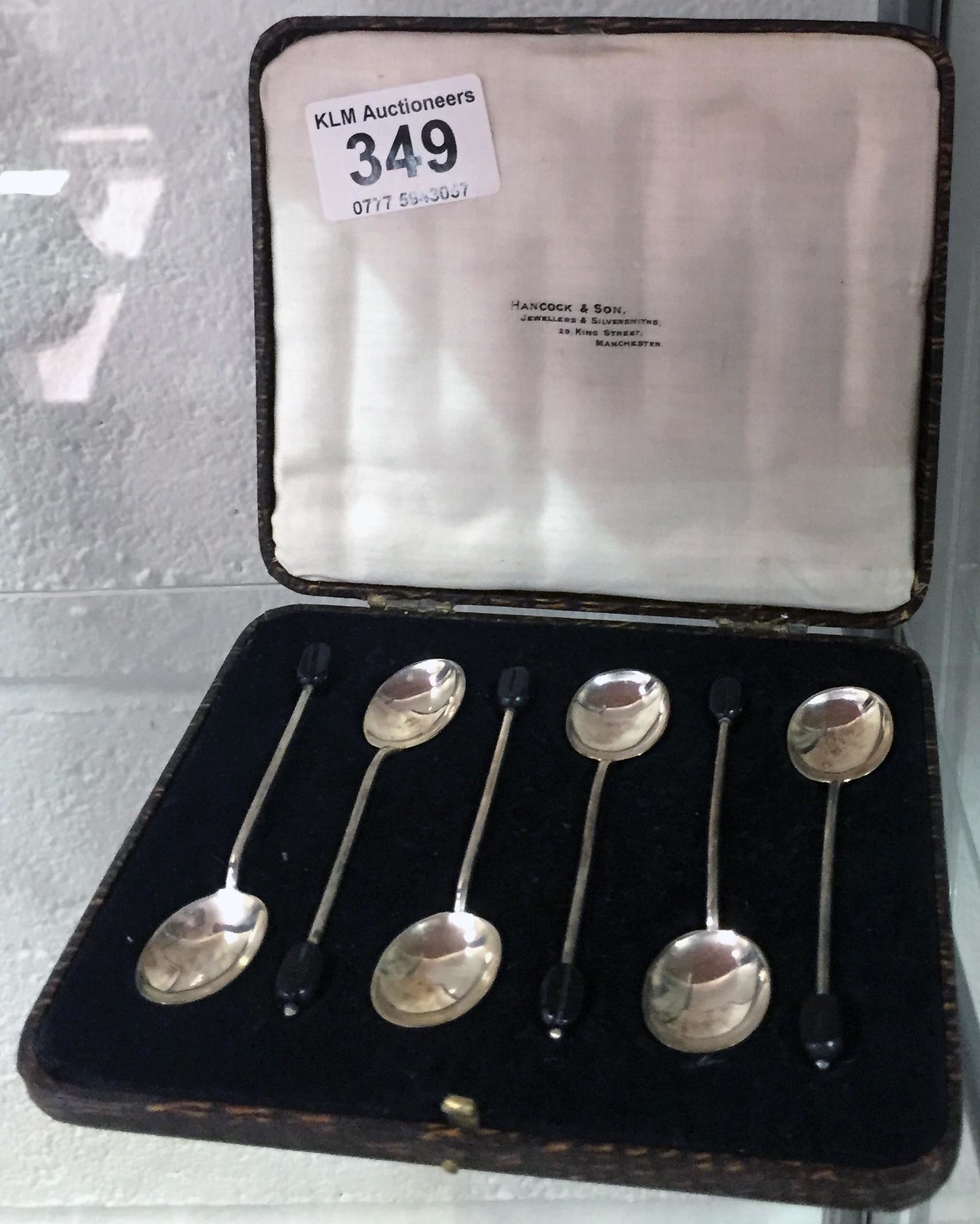This black and white photograph, likely taken through glass given the visible reflections, depicts an open, clamshell-style wooden silverware case propped ajar against a white stucco wall. The interior features a plush white satin lining on the lid and a black velvet base with cutouts that securely nestle six finely polished, wide soup spoons. Notably, the spoons, which could be sterling silver, have very thin stems ending in round, black, coffee-bean-like knobs. The age of the wooden case suggests the silverware is antique. A sticker on the top left of the inner lid reads "KLM Auctioneers 349," indicating the item is up for auction.